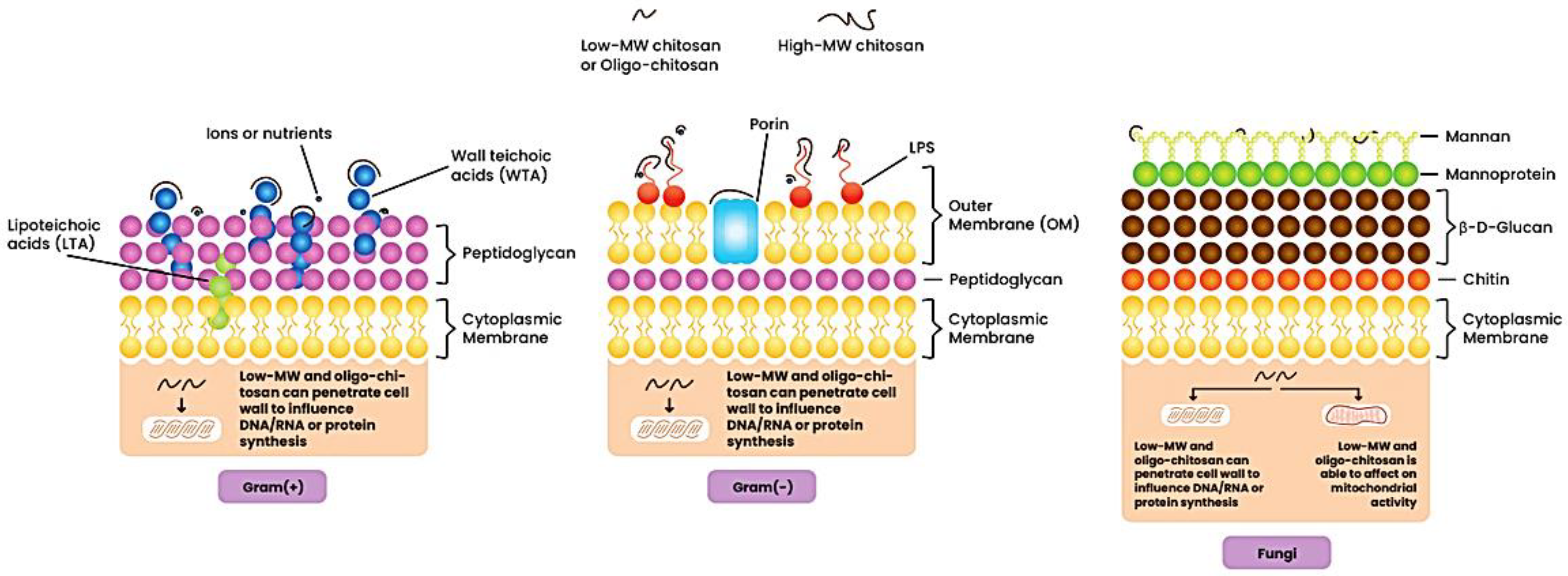The scientific illustration features detailed labels and color-coded sections that depict various biological components and their interactions with chitosan. At the top left, a small black squiggle labeled "low MW Chitosan" or "Oligo Chitosan" appears, while to its right, a longer squiggle is labeled "high MW Chitosan."

Below these labels, the illustration is divided into three sections, each showcasing different cell components with a peach-colored base. The left section includes blue, purple, and yellow elements representing lipoteichoic acid (LTA), wall teichoic acids (WTA), peptidoglycan, and the cytoplasmic membrane, identified as Gram-positive bacteria. This section emphasizes that low MW and Oligo Chitosan can penetrate cell walls to influence DNA, RNA, or protein synthesis.

The middle section features red, yellow, and pink elements for porin, lipopolysaccharides (LPS), an outer membrane, peptidoglycan, and a cytoplasmic membrane indicative of Gram-negative bacteria. Here too, it is noted that low MW and Oligo Chitosan can penetrate cell walls to affect DNA, RNA, or protein synthesis.

The right section displays green, brown, red, and yellow elements representing mannan, manoprotein, peptidoglycan, and a cytoplasmic membrane associated with fungi. This section notes that low MW and Oligo Chitosan can penetrate cell walls, influencing DNA, RNA, or protein synthesis, and can also affect mitochondrial activity.

The illustration uses a mix of black text and various colored shapes like balls and squares to indicate different biological structures and their interactions with chitosan.